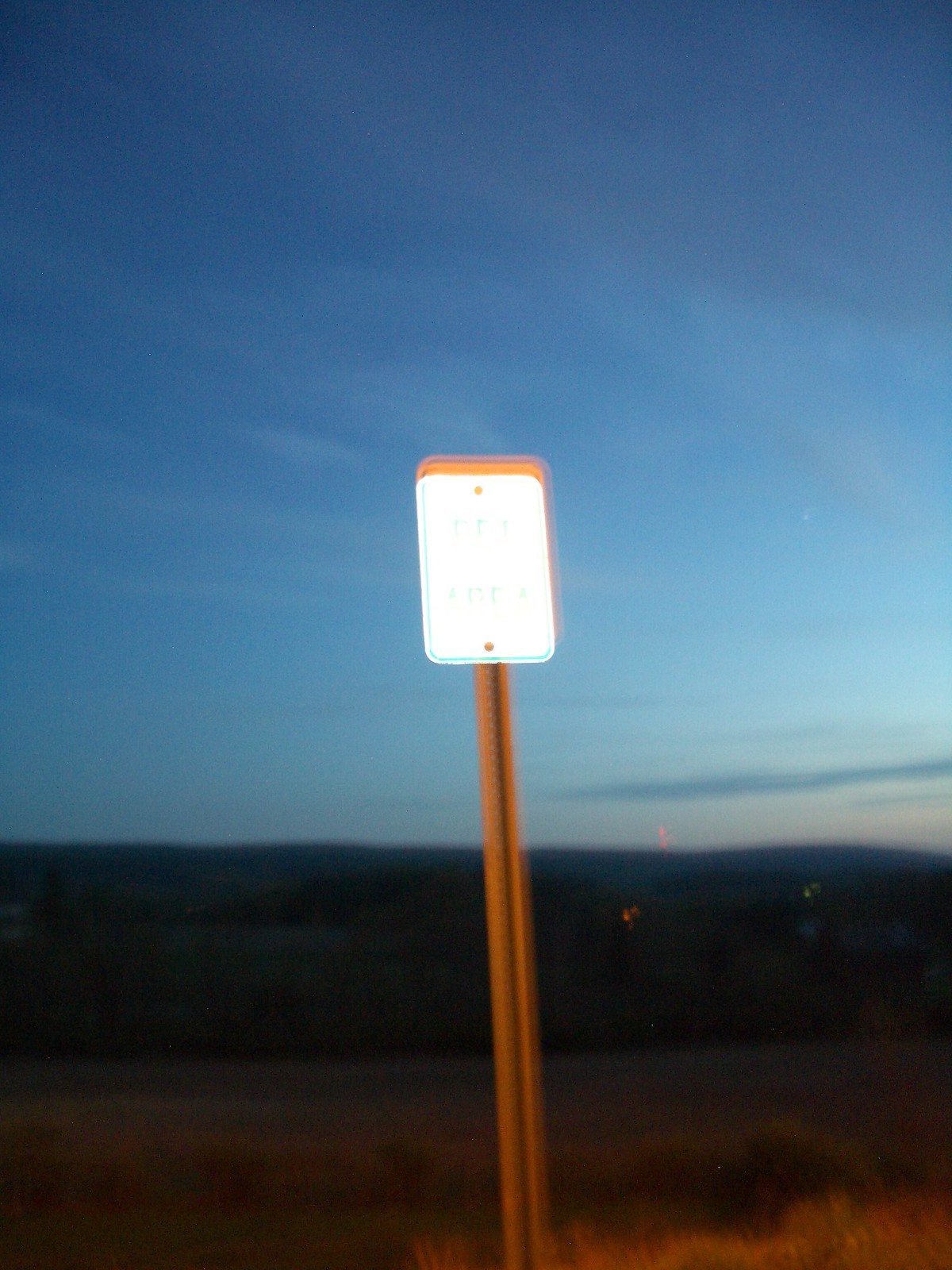This photograph, captured in the evening, showcases a white rectangular road sign mounted on a long, perforated metal post. The scene is set in a deserted, possibly desert-like area with flat, dark terrain, and faint reddish-colored brush visible towards the lower right corner of the image. The sky, transitioning from deep blue at the top to a lighter shade near the horizon, retains a hint of sunlight and is adorned with wispy white clouds. The sign, seemingly illuminated by direct light, appears blurred or double-exposed, making its text nearly illegible, though it suggests two words in blue capital letters. The overall setting exudes a tranquil yet mysterious twilight ambiance.